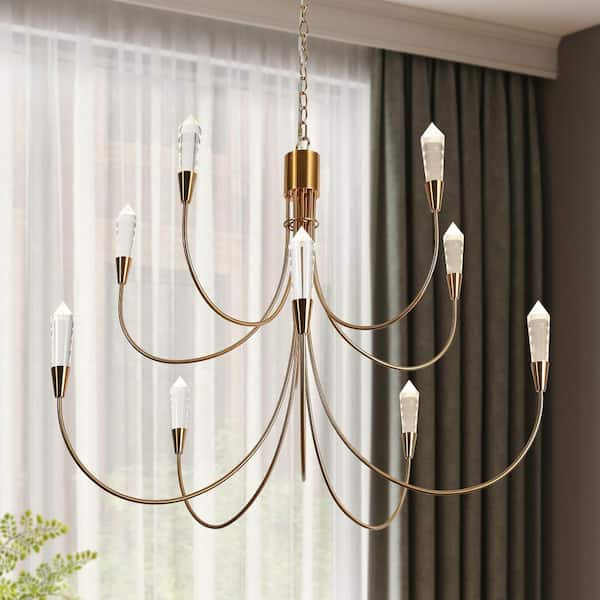The close-up photograph captures an elegant, somewhat modern chandelier featuring a gold or copper-colored chain hanging from the ceiling, culminating in a cylindrical base from which multiple thin, looped arms extend. There are nine arms in total, each supporting a conical, white crystal-like light fixture, enhancing the chandelier's sleek aesthetic. The image is taken indoors under artificial lighting, ensuring the chandelier is well-lit, well-framed, and in focus, making it the central focal point.

In the lower corners of the image, green leaves from a small house plant add a touch of nature. The background showcases a large window adorned with a combination of sheer white, lacy curtains and heavier, solid gray or dark brown drapes. The room’s decor is further characterized by bone-colored wood molding, a gray wall, and a white ceiling. Overall, this vibrant and detailed photograph conveys a sophisticated yet modern home decor ambiance, likely intended for a home decor website, blog, or magazine.